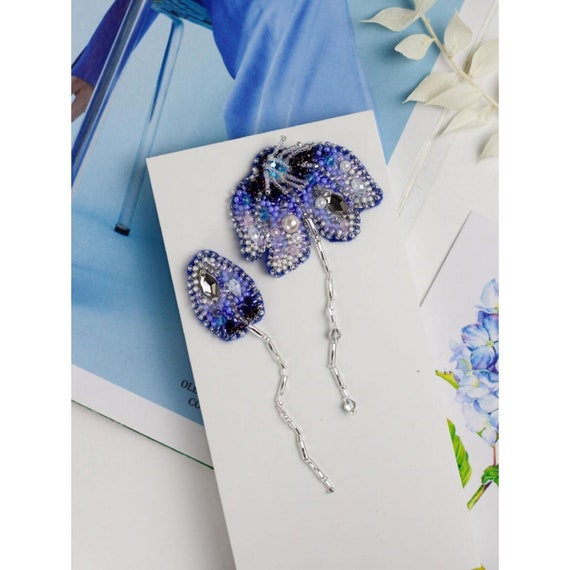This photograph captures a detailed display of two intricately beaded decorations arranged on a white cardstock. The left decoration, reminiscent of a tadpole, features a blue beaded top complemented by a long silver beaded tail. The decoration on the right, resembling a butterfly or umbrella, showcases a striking combination of blue, purple, and white beads with an ornate black beaded top and a similar silver beaded tail. Both beaded items are adorned with pearl-like white beads scattered throughout their designs. The background includes an array of additional cards, one depicting a person seated in a chair wearing blue pants, another featuring blue flowers, and a sketch of white leaves in the top right corner, adding layers of visual interest to the scene. Scattered flower petals add a delicate touch to the overall composition.